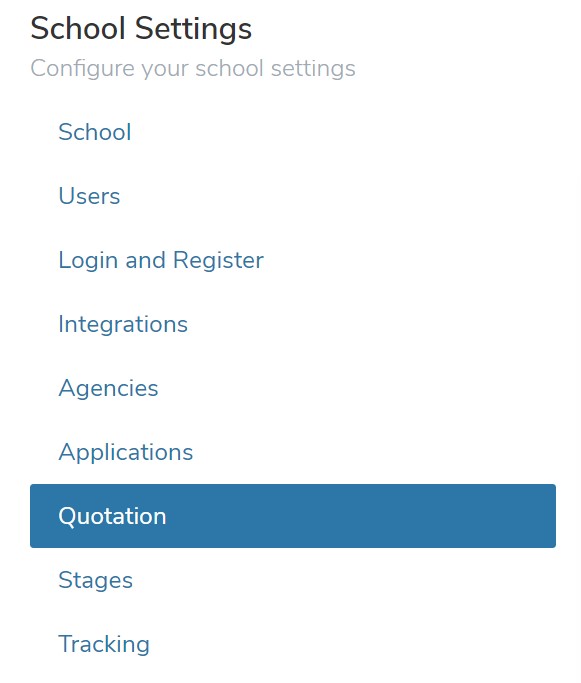On a white background, the image features a school management system interface. At the top, in gray text, it prompts users to "Configure Your School Settings." Below this, in blue text, options are provided for "Schools or School," "Users," "Log In," "Register," "Integrations," "Agencies," and "Applications." At the bottom, a blue rectangle contains the word "Quotation" written in white.